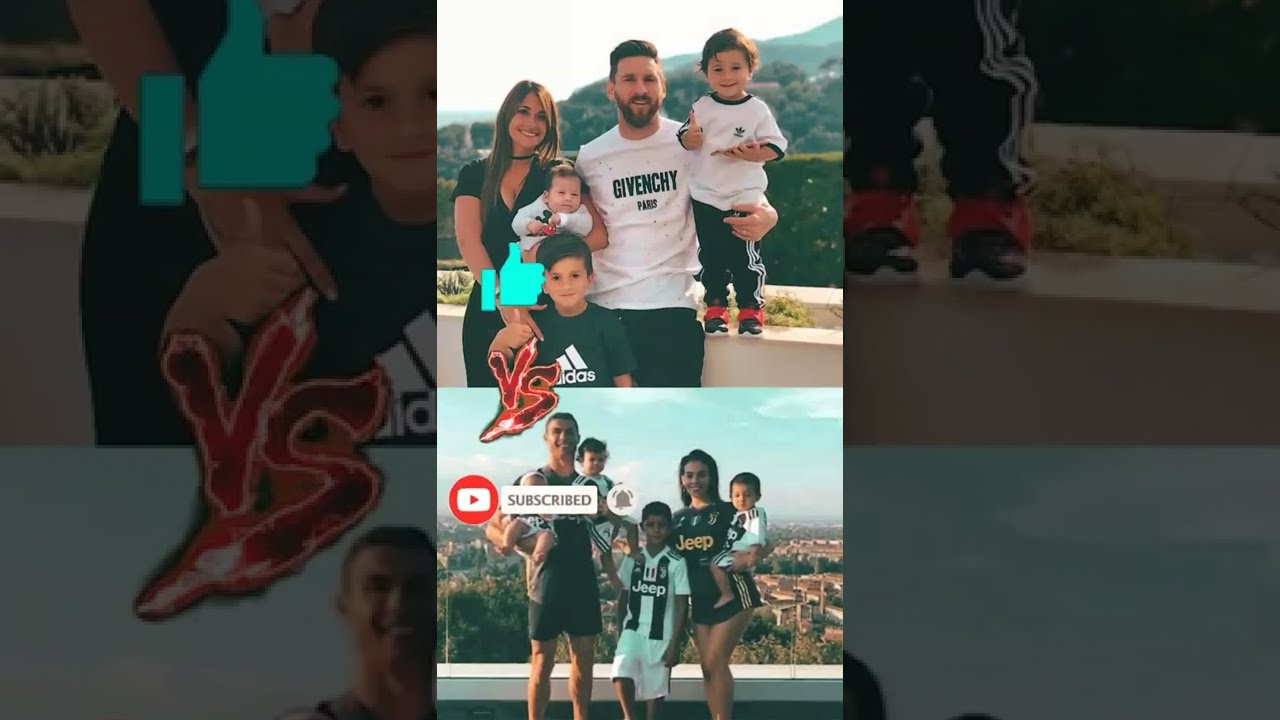The image features a split-screen composition with two family photos, one above the other, set against diverse backgrounds showcasing hills, mountains, cityscapes, and skies. The top image captures a woman with her spouse, who wears a Givenchy shirt, along with their three children: two young boys and an infant. The bottom image depicts another family, possibly different, consisting of a man and a woman and their three children, also two young boys and an infant, wearing soccer jerseys from brands like Adidas and Jeep. These families are dressed in colors including black, white, gray, blue, green, red, light blue, and brown. The images suggest a competitive context with the word "versus" in red and a thumbs-up emoji on the top photo, while the bottom photo includes a YouTube "subscribed" button with a bell. The backgrounds of both main images feature a blown-up, zoomed-in, darker version of the same scenes, adding depth and context. These visual cues imply that the families may be engaging in a friendly soccer match or similar event, with the occasion being shared on YouTube, highlighting the athletic and familial spirit.